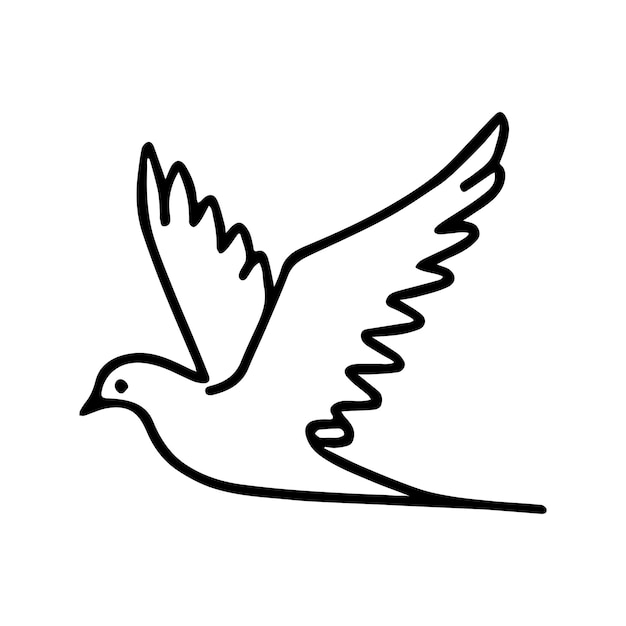This image features a minimalist, side-view sketch of a dove in mid-flight. The dove is depicted using thick, bold black lines that outline its form against a plain white background. The head of the bird faces to the left, showing a beak and a single dot for the eye. Both wings are positioned upward, with one wing slightly more tilted, suggesting movement. The body of the dove tapers to a sharp tail, represented by precise black lines. The simplicity of the linework and the absence of internal details emphasize the bird’s minimalistic and elegant design.